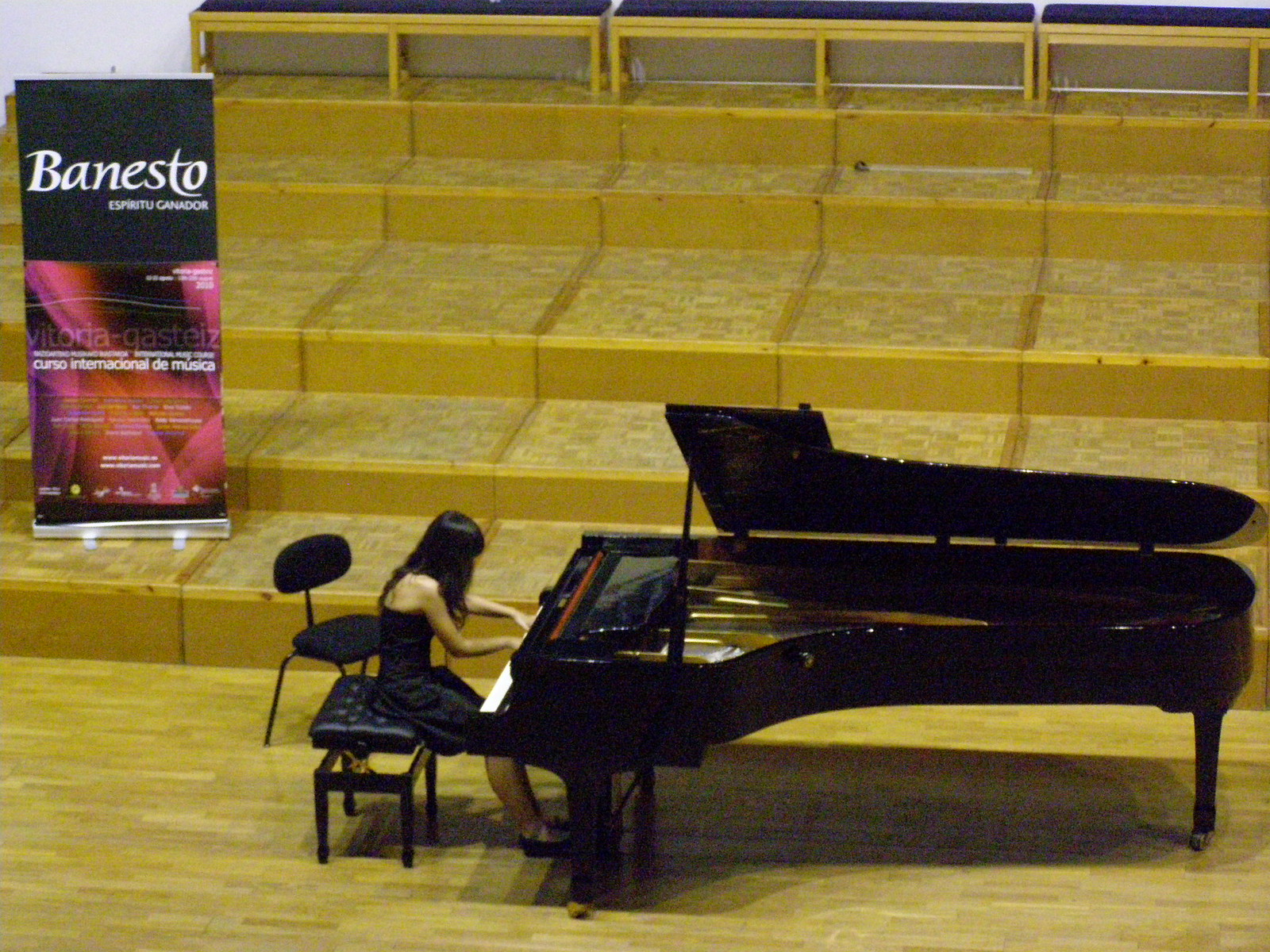The image captures a detailed indoor scene featuring a live musical performance on a terraced wood parquet stage with a light brown hardwood finish. Central to the image is a grand black piano with the top open, its elegant, elongated form dominating the scene. Seated at the piano is a slim woman with long, dark hair, immaculately dressed in a black dress complemented by black shoes. She sits on a four-legged, padded black piano bench and leans forward, engaged in playing the piano keys. To her right stands a black chair. On the upper left quadrant of the background, there is a banner sign with a top section that has a black background with white text reading "B-A-N-E-S-T-O." Below this is a red shadowed design with additional white text. The entire scene is encapsulated by an atmosphere that appears to be part of a stage performance, indicating an indoor setting but with no visible indication of the time of day. The colors in the image include black, white, pink, tan, and brown.